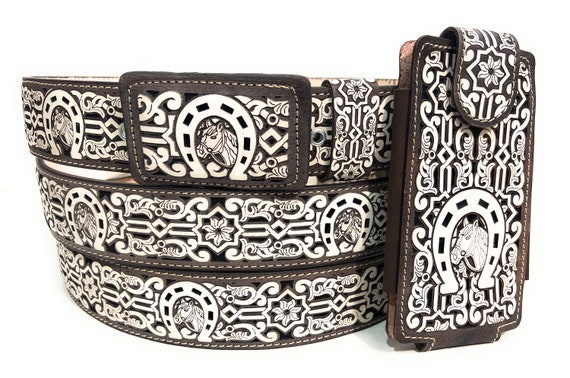This photograph showcases a collection of intricately designed leather items, prominently featuring a coiled belt and a wallet or phone case. Central to the image, the dark brown leather belt is artistically arranged in overlapping layers, resembling a coiled snake. Both the belt and the wallet are adorned with detailed white stitching and feature a variety of embossed and painted designs. These designs include a horseshoe motif encircling a horse's head, and additional decorative elements such as floral patterns and triangular, Viking-like accents. The wallet, standing upright next to the belt, displays a strap closure, likely secured with Velcro. The color palette of the items includes dark brown leather with contrasting white accents, set against a predominantly brown background. The craftsmanship and thematic elements of these leather pieces underscore their cowboy-inspired aesthetic.